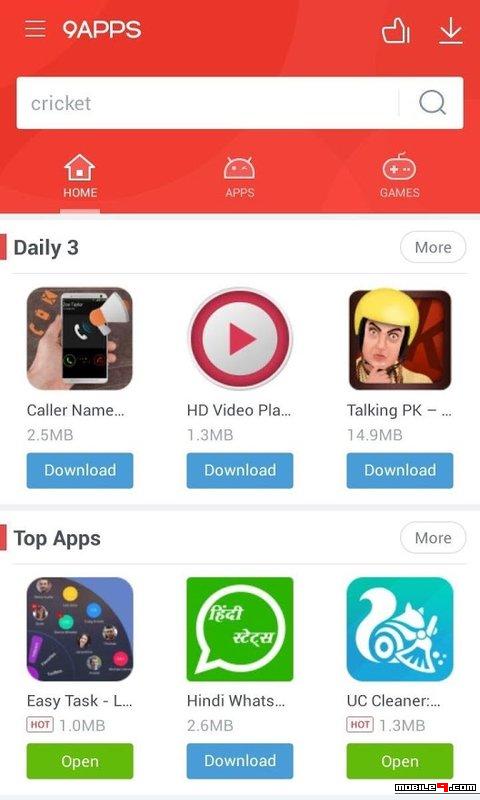The image is a screenshot of an app or website interface. In the top third of the screen, there is a prominently colored red block. Situated in the top left corner, there are three white horizontal lines representing the menu icon. Next to the menu icon, the text "9apps" appears in white print. On the right-hand side of this red block, two icons are visible: a thumbs-up symbol and a downward-pointing arrow icon indicating download functionality.

Beneath this red block, a search bar is present with the term "cricket" entered into it. Directly below the search bar, there are three tabs: "Home," "Apps," and "Games," with the "Home" tab currently selected.

In the mid-third of the screen, there is a section labeled "Daily 3," which features three app icons in a row:
- The first icon depicts a hand holding a phone with a megaphone above it, labeled "Caller Name."
- The second icon is a red-bordered circle with a white interior containing a right-pointing triangle, representing a play button, labeled "HD Video Player."
- The third icon shows a person wearing a yellow helmet, labeled "Talking PK."

Each of these apps has a download button located beneath its icon.

Moving towards the bottom of the screen, a section titled "Top Apps" displays three more app icons in a row:
- The first app, "EasyTask," shows several small icons and an "Open" button located below it.
- The middle icon is green with a white speech bubble containing some text, representing "Hindi Watts," and it has a download button below it.
- The last app features a cute squirrel holding a broom, labeled "UC Cleaner," with an "Open" button beneath it.

This detailed layout vividly describes the various components and icons present on the interface, capturing the essence of the content portrayed in the original image.